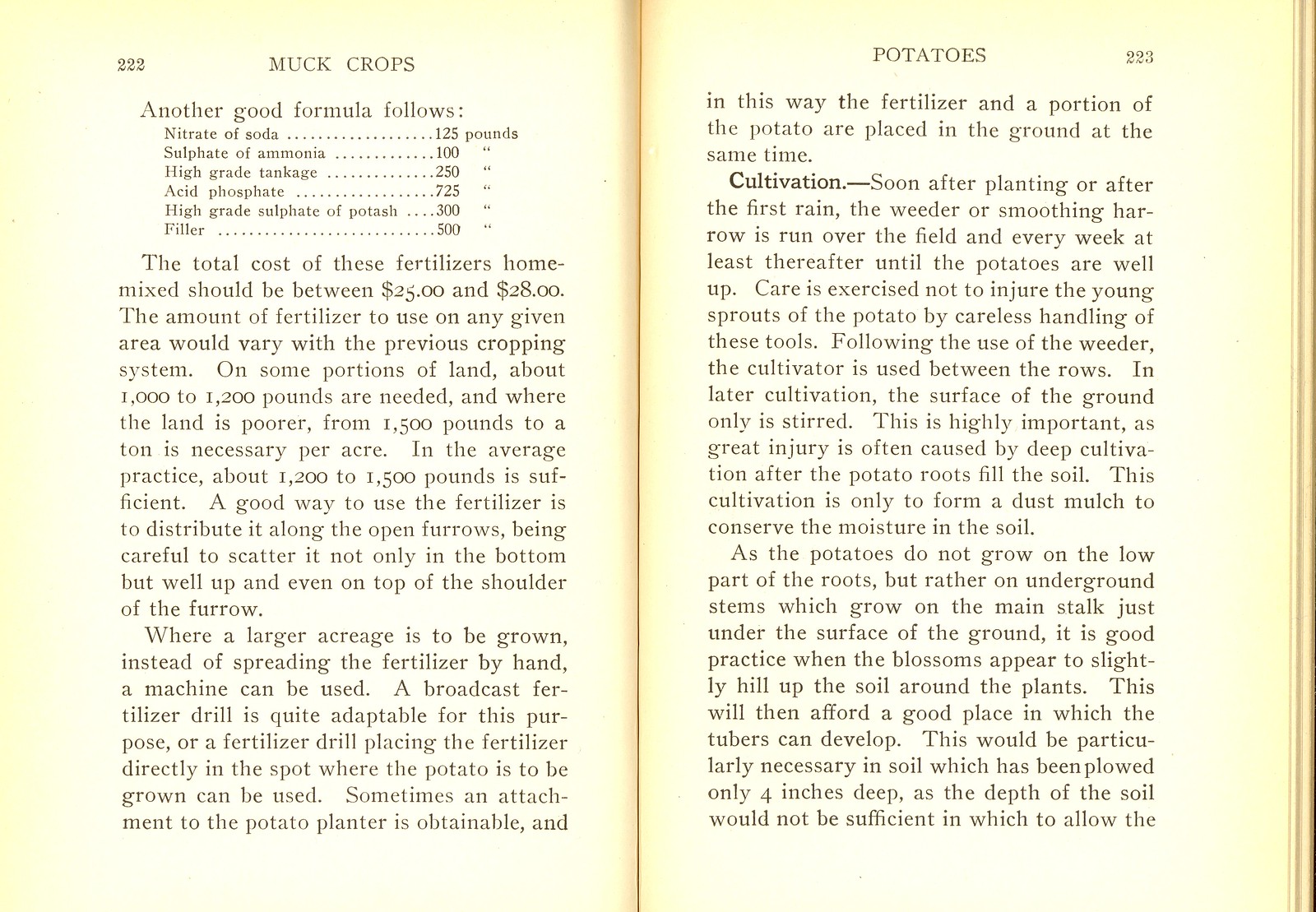This image depicts two pages from a book, specifically pages 222 and 223. On page 222, titled "Crops," there is detailed information about fertilizer formulas and usage. The recommended formula includes 125 pounds of nitrate of soda, 100 pounds of sulfate of ammonia, 250 pounds of high-grade tankage, 725 pounds of acid phosphate, 300 pounds of high-grade sulfate of potash, and 500 pounds of filler. The total cost of this home-mixed fertilizer should range between $25 and $28. The amount of fertilizer needed varies based on previous crop cycles. Generally, 1,200 to 1,500 pounds per acre is recommended for average conditions. Fertilizer should be distributed in open furrows, either by hand or using a broadcast fertilizer drill or a specialized fertilizer drill. For larger areas, machinery is preferred to ensure even distribution.

Page 223 continues from the previous page under the heading "Potatoes." It describes the process of planting and cultivating potatoes. Fertilizer and a portion of the potato are placed in the furrow simultaneously. After planting or the first rain, a weeder or smoothing harrow is run over the field weekly. Care must be taken not to damage young sprouts. Following the weeder, a cultivator is used between rows, ensuring only surface soil is stirred to create a dust mulch that conserves moisture, essential for potato growth. Potatoes develop on underground stems rather than on deep roots. When blossoms appear, soil should be hilled around the plants to provide space for tuber development, particularly in fields plowed to a shallow depth.